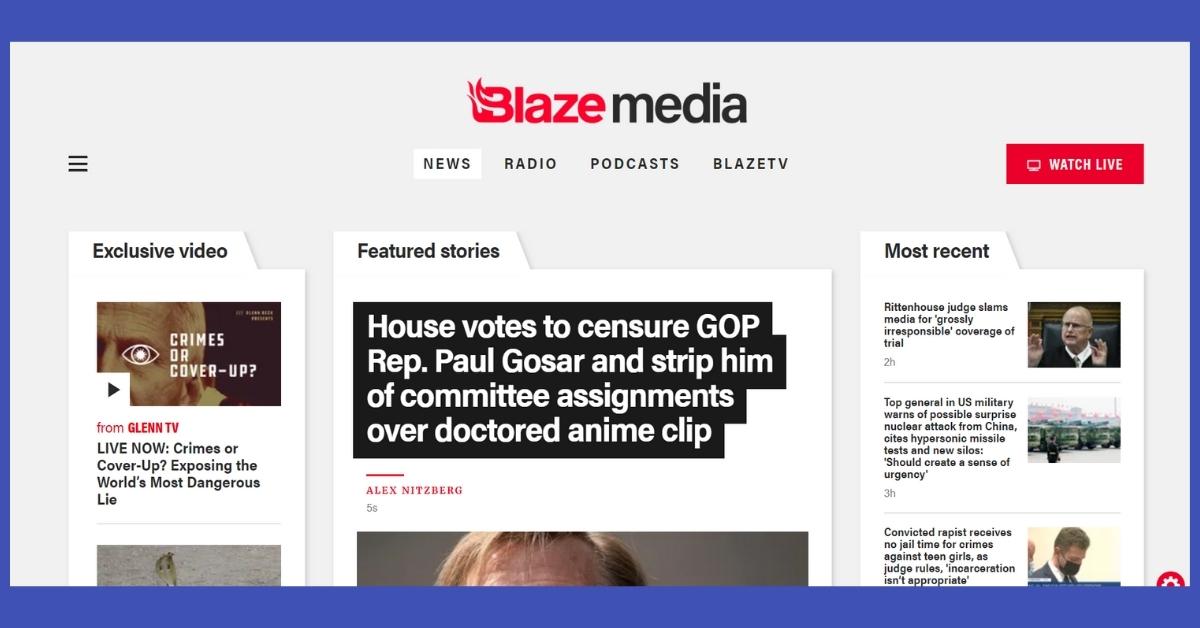The image captures the Blaze Media website, featuring a prominent logo with "Blaze" in bold red letters and a flame emerging from the "B." Directly below the logo, the navigation menu lists options: News, Radio, Podcasts, and Blaze TV, indicating a diverse media platform. The highlighted section is News, accompanied by tabs such as "Exclusive Video" and "Crime to Cover Up," the latter having a play option and described as "Exposing the World's Most Dangerous Lie." 

At the top right, a settings icon with three horizontal lines is visible. The "Feature Stories" section prominently displays a reversed-print headline about a recent update, "House," timestamped five seconds ago, featuring a cropped image showing a person's forehead and hair. 

An option to "Watch Live" is positioned above other recent articles, including:
1. "The Rittenhouse Judge Slams the Media for Irresponsible Coverage of Trial."
2. "The Top Journal is U.S. Military."
3. "Convicted Rapist Received No Jail Time."

A gear icon is located at the bottom right, likely for additional settings. The entire Blaze Media webpage is bordered by a distinctive blue frame.